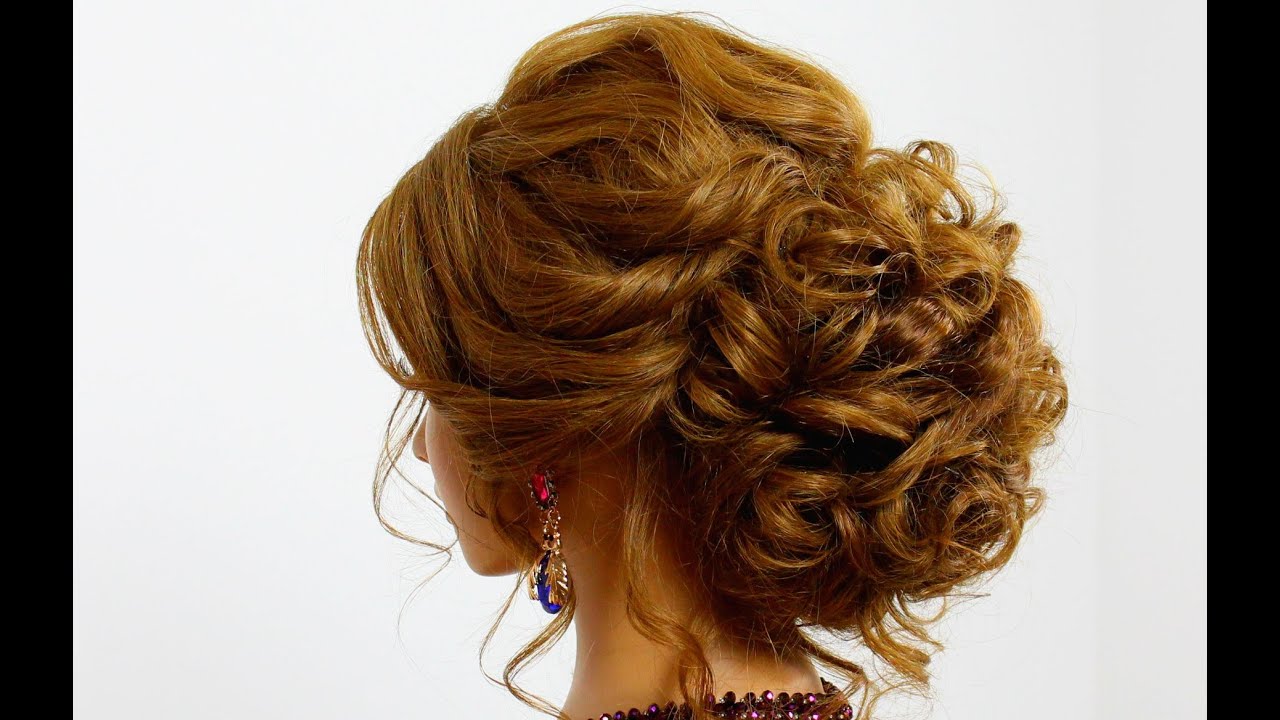The image features a detailed profile view of a woman’s head and neck, set against a light gray background framed by vertical black bars on either side. The woman is turned slightly to the left, showing the back of her head and just a hint of her facial features, including her nose and lips. Her hair, a rich auburn or reddish-brown color, is intricately styled into a voluminous, ornate bun composed of numerous twists and curls. Some loose, stringy hairs fall around her face and neck. She adorns an elaborate earring on her left ear, which features a red gem at the top, small gold hoops, and two gold leaves encircling a large blue gemstone, resembling a cicada. Just visible at the base of her neck is the top of a sequined purple garment.